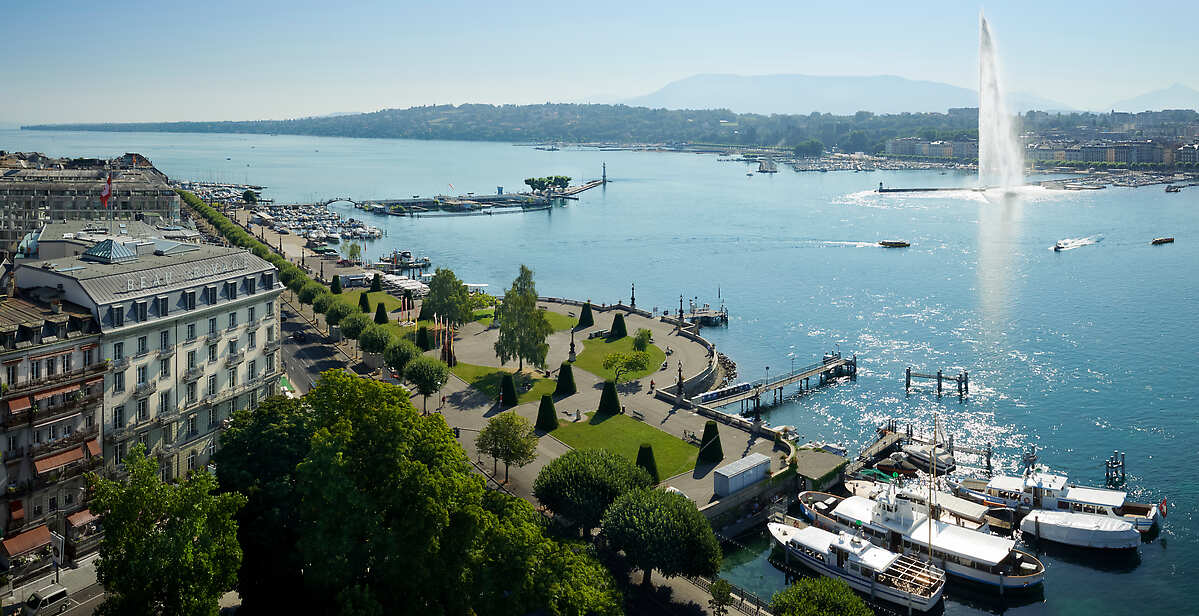This aerial photograph captures a picturesque harbour town, bathed in sunlight on a summer day. In the lower left, quaint paths weave through grassy areas and past historic shops with old-fashioned awnings, giving the scene a nostalgic charm. People are scattered leisurely along the harbour walls, which curve protectively around a collection of moored boats of various sizes.

Dominating the left side of the image, a waterside hotel, possibly a refurbished classic, stands with elegance against a backdrop of lush trees. A jetty extends out into the shimmering, dark blue water, adding depth to the bustling harbour scene. The right side of the image shifts focus to a larger dock, where bigger boats are tethered.

Across the river that bisects the town, another cityscape rises, marked by verdant greenery and perhaps unnaturally perfect pyramid-shaped structures, suggesting a possibly AI-generated enhancement. A striking spectacle in the upper right corner draws immediate attention—a powerful jet of water shoots skyward, resembling a fountain or a mystical water spout, casting a surreal touch to the historical ambiance.

In the distance, a green mesa overlooks the bay, completing the serene yet vibrant tableau of this coastal paradise.